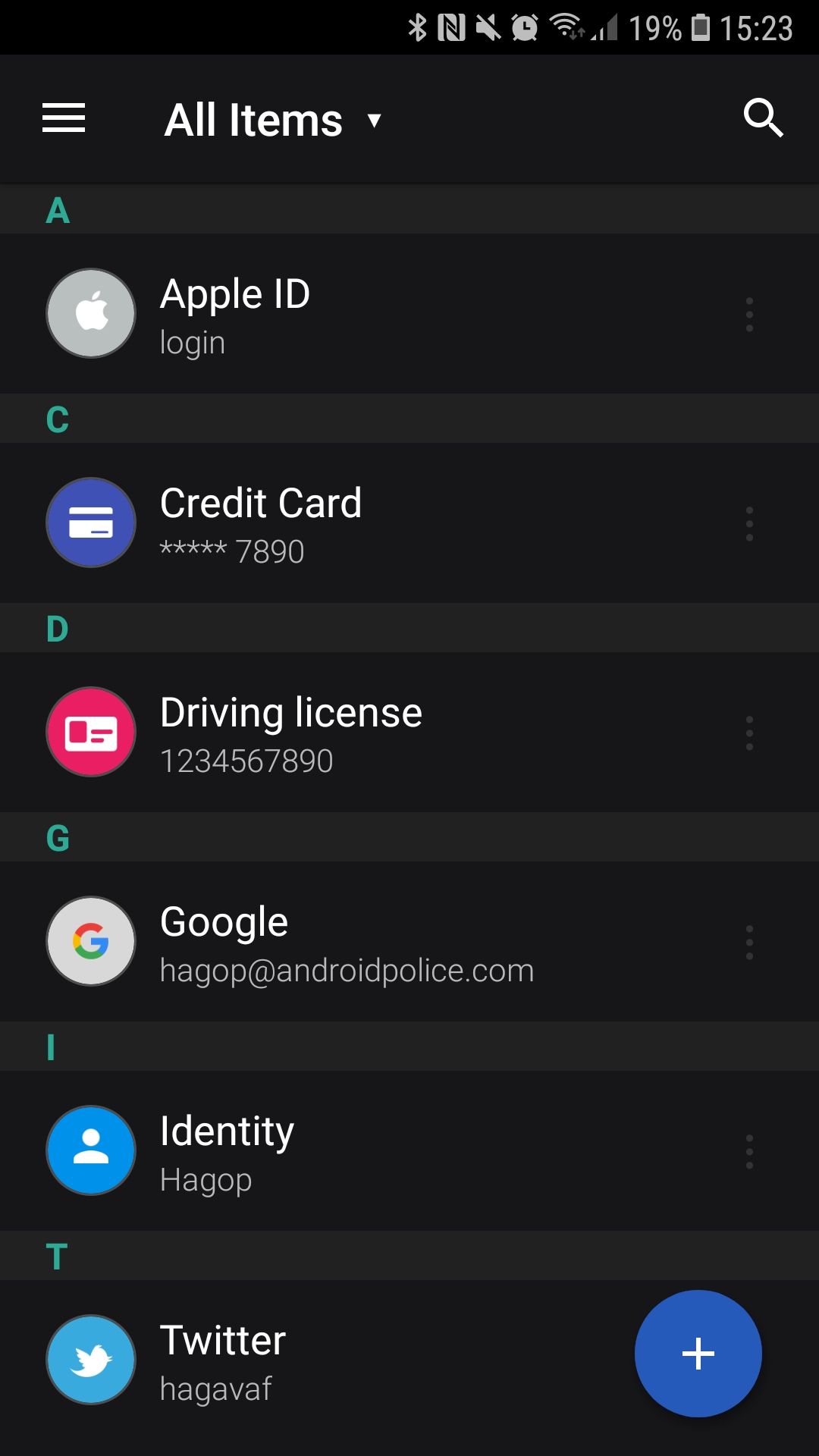The image is a vertical rectangle with a predominantly black background, seemingly captured from a smartphone display. At the very top center, a series of standard phone icons are visible: a Bluetooth symbol, a speaker icon indicating silence mode, an alarm clock, a fully filled Wi-Fi signal, a cell signal with two bars, a battery icon displaying 19% charge, and the time, marked as 15:23. Directly beneath these icons, there's a navigation bar featuring three icons: a hamburger menu on the left, an "All Items" dropdown arrow in the middle, and a search icon on the right.

Further down, the display shows various categories, each accompanied by a distinct icon on their left. The categories listed are: "Apple ID," which has an Apple logo; "Credit Card," with a credit card icon; "Driving License," represented by an icon resembling a driver's license; "Google," with the Google 'G' icon; and "Identity," marked by an icon depicting a person's silhouette.